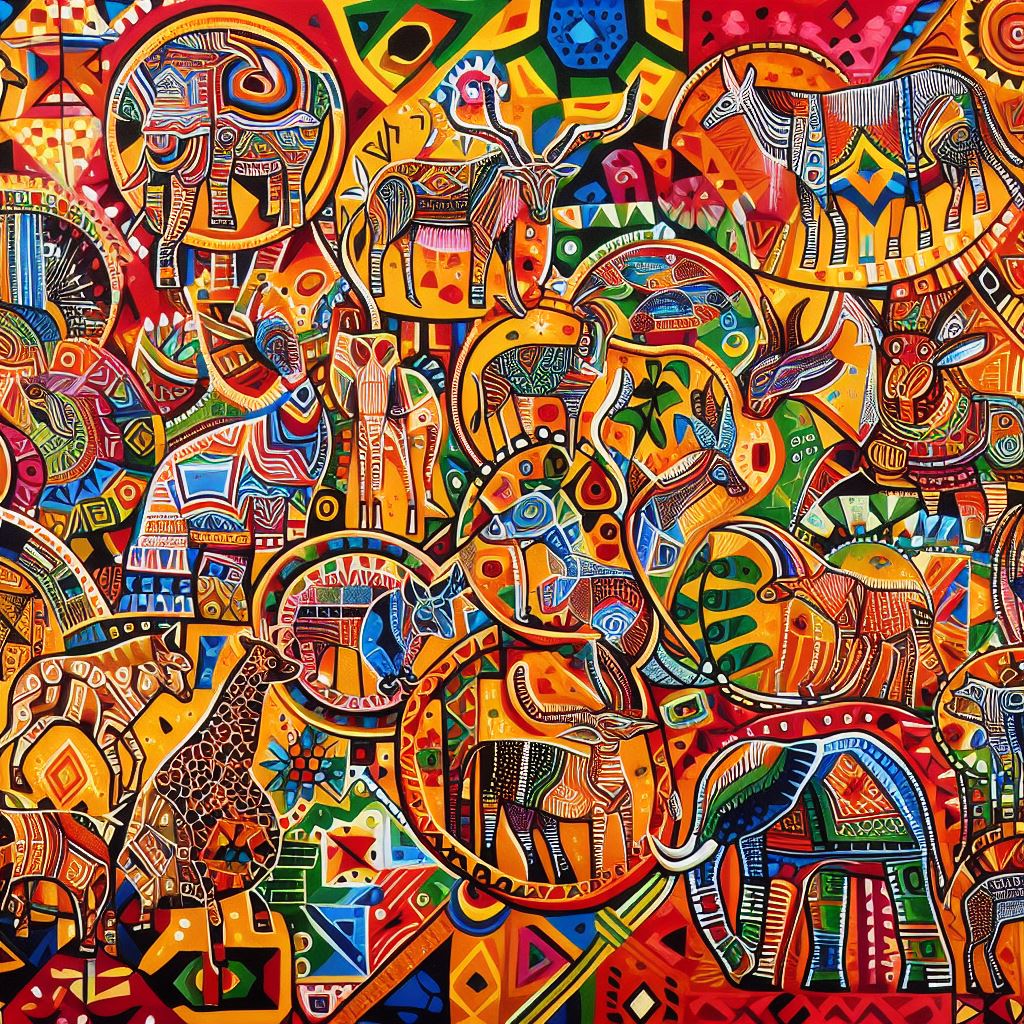This vibrant Afrocentric painting captivates with its rich palette of colors, including striking hues of blue, green, orange, yellow, black, white, and red. The intricate patterns of lines, circles, dots, and zigzags create a dynamic backdrop for an array of African wildlife. Scattered across the canvas are meticulously depicted animals such as an antelope with prominent antlers, a tall and elegant giraffe, a distinctive zebra, and majestic elephants. Each creature's gaze varies, with some looking to the right, others to the left, and a few seemingly staring directly at the viewer, inviting them into the lively, animated world of the painting.